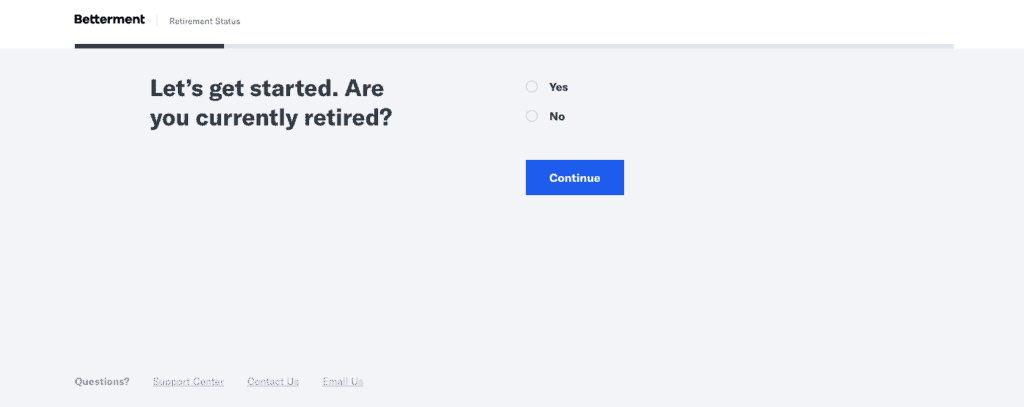This screenshot from Betterment focuses on the user interface for assessing retirement status. The layout is exceptionally clean and modern, utilizing a contemporary, high-tech design theme. At the top of the screen, a prompt reads, "Let's get started. Are you currently retired?" Beneath the prompt are two prominent buttons labeled "Yes" and "No" for users to indicate their retirement status. 

Once a selection is made, a blue button with white text appears, labeled "Continue," guiding users to the next step. The bottom section features a support area with clickable options, including "Questions," "Support Center," "Contact Us," and an "Email Us" button, acknowledging the complexity of retirement planning and offering various means of contacting Betterment for assistance.

The color palette combines light gray backgrounds with dark text, creating a visually appealing and easy-to-read interface. This thoughtful use of colors and layout can enhance user experience significantly. The overall design is both clean and functional, ensuring users can navigate the retirement planning process with ease.